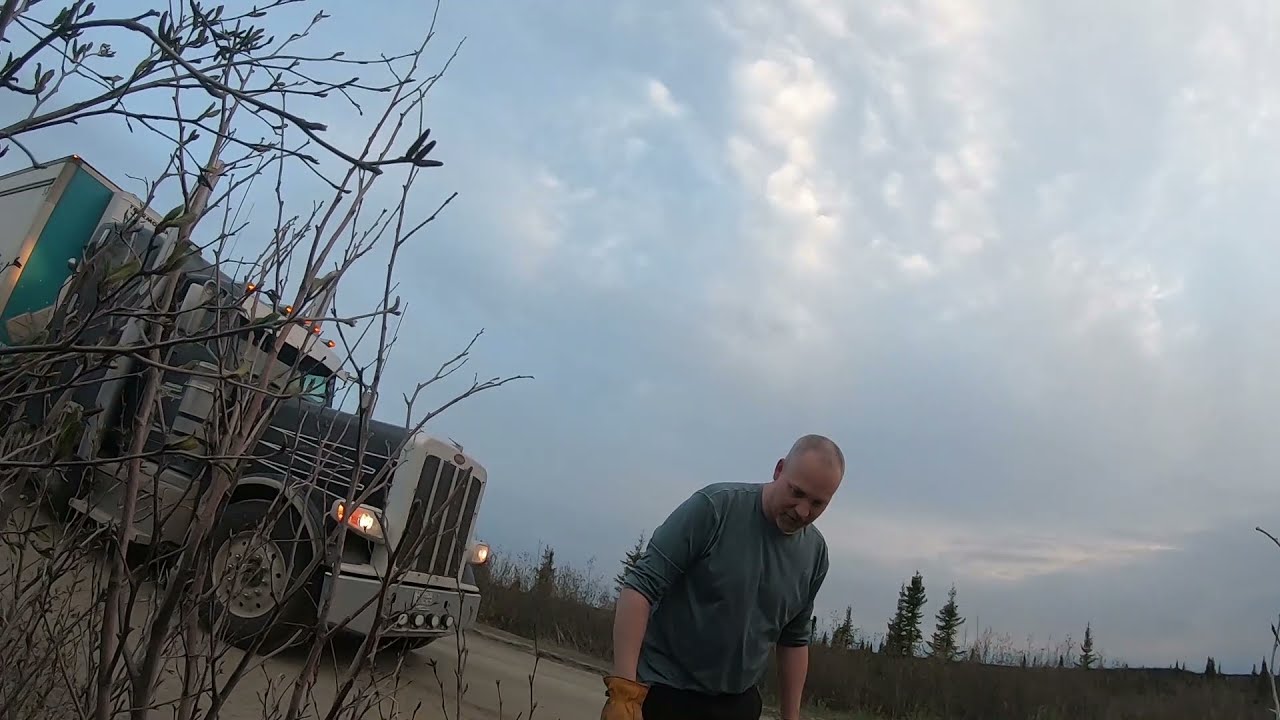The full-color photograph, taken outdoors on an overcast day, prominently features a cloudy sky dominating most of the image. Towards the lower part of the picture, a stretch of trees, including evergreens and leafless branches, outline the horizon. In the foreground, standing among some barren bushes and twigs, is a 40-ish year old man wearing a green shirt with rolled-up sleeves and brown work gloves. He is balding and appears to be intently searching for something on the ground. Nearby, a large semi-truck with its headlights on is parked along the roadside, partially obscured by the bushes. It is likely the man is the truck driver, possibly looking for a part or object that might have fallen. The diffused light from the overcast sky gives the scene a somewhat dim appearance, suggesting an uncertain time of day.